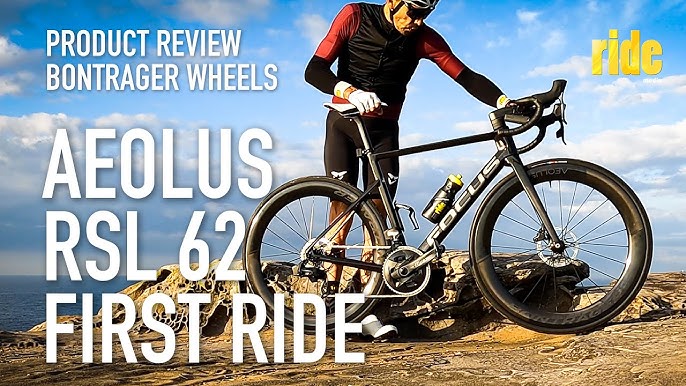In this detailed rectangular photograph, a product review for the Bontrager Wheels Aeolus RSL 62 First Ride is illustrated. Set against a backdrop of a hilltop with brown rocks and an expansive sky, a cyclist is prominently featured. The rider, donning a red and black long-sleeve shirt, black pants, and large visor-like sunglasses, stands beside a black-framed mountain bike labeled "Focus," with one hand on the seat and the other on the handlebars. The bike, equipped with thick tubes and a water bottle holder, is positioned to the right. The cyclist also wears a white helmet and specialized shoes. Text is displayed on the left side of the image, reading, "PRODUCT REVIEW BONT RAGER WHEELS" in all caps and "Aeolus RSL 62 FIRST RIDE" in larger font. Additionally, the word "ride" appears at the top right in yellow font, emphasizing the review's focus on the cycling experience.